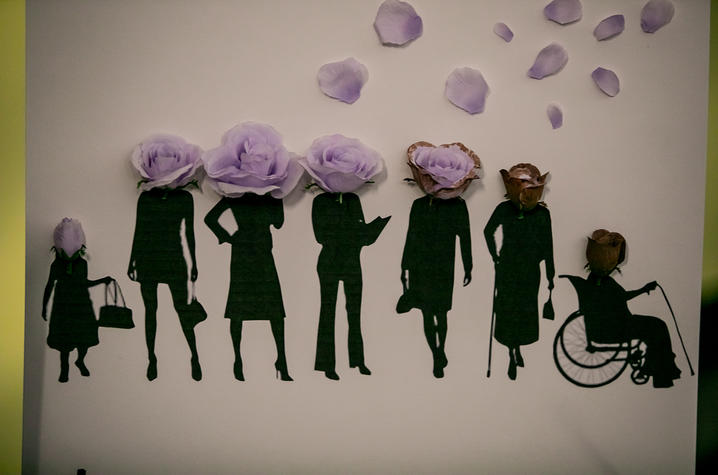The image is an artistic depiction on a white background featuring seven black silhouettes arranged in a row, representing various stages of life and roles of women. The figures lack human heads and faces, instead, they are topped with purple rose flowers. Starting from the left, the first figure is a child holding a purse, while the remaining silhouettes portray adult women. Among these adults, two women carry handbags, one positioned towards the far left and another towards the far right. Additionally, one of the adult figures near the center holds a cane. On the farthest right, an individual in a wheelchair also holds a cane and sports a head covering. Above the figures, scattered flower petals adorn the scene, adding an ethereal, delicate touch to the tableau. The entire composition is rendered in the style of cut-out black construction paper silhouettes, setting a distinct contrast against the stark white background.